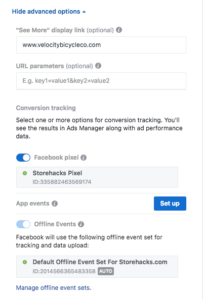The image features a user interface displayed against a clean, white background. A thin, light gray vertical line runs down the far right side of the image, extending from the top to the bottom. Positioned at the top left in blue text, the phrase "Hide advanced options" can be seen. Directly beneath it, in gray text, it reads "See more display link optional."

Below these lines of text, there is a text box containing the URL "www.velocitybicycleco.com." Underneath this, the phrase "URL parameters optional" can be observed, followed by another text box, which contains some unreadable, blurry text.

Continuing down the image, the heading "Conversion Tracking" is displayed, along with a subheading that instructs: "Select one or more options for conversion tracking. You'll see the results in Ads Manager along with ad performance data." Directly below, there is a toggle bar set to the right, indicating it is active, and colored blue. This toggle is labeled "Facebook Pixel," accompanied by a series of numbers underneath.

Adjacent to the "Facebook Pixel" section, there is a blue button labeled "Setup." Beside it, the words "App Events" are displayed next to a small gray circle, indicating this option is unselected or inactive.